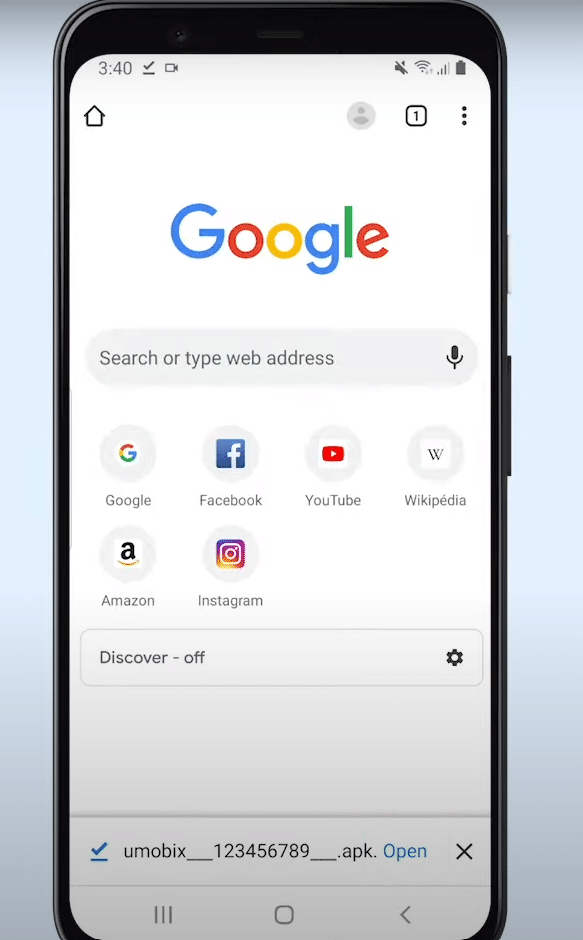The image captures a Samsung phone displaying the Google search page. The phone, showcased against a light blue backdrop with subtle grey corners, is characterized by its dark grey or black hue. On the screen, the Google search page is prominently white. At the top left, the home button is visible, while the top right features the user profile button, tabs button, and a small menu icon. Below these icons, the Google logo is centrally placed with a search bar beneath it, which includes a microphone icon on its right side for voice search functionality.

Under the search bar, there is a series of bookmarks, in order: Google, Facebook, YouTube, Wikipedia, Amazon, and Instagram. Below these bookmarks, a small bar displays the message "Discover Off" with a settings icon situated to the right. Towards the bottom of the screen, a small pop-up indicates a recent download completion, featuring a checkmark, the file name (an APK file), and an “Open” button. Finally, at the very bottom of the image, the Samsung phone’s physical buttons are visible.